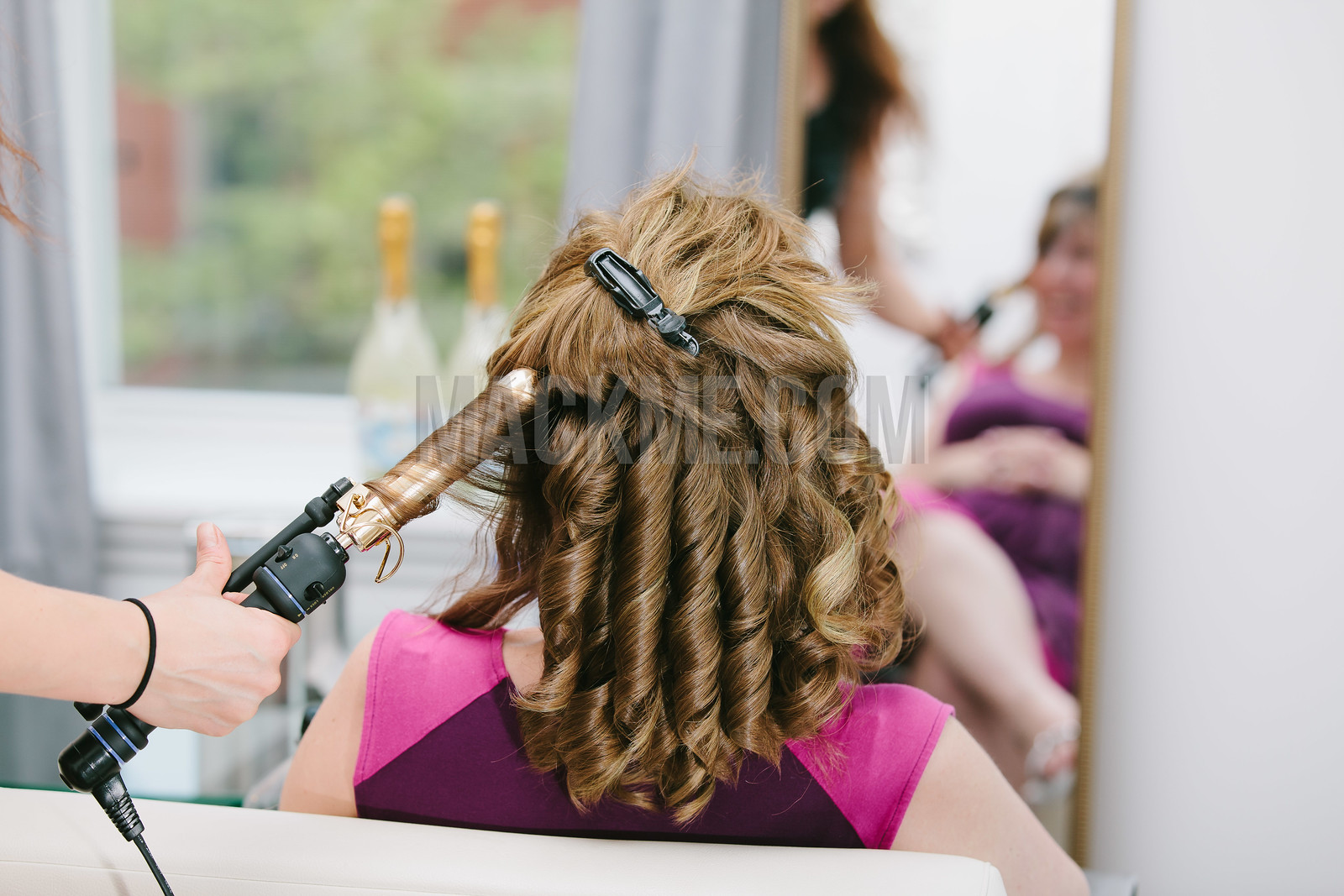This photograph captures a detailed scene of a woman with shoulder-length brown hair being styled into dramatic curls at a salon. She is seated in a white chair, wearing a short-sleeved blouse that appears to be a mix of pink and dark purple. Most of her hair is already styled into long, flowing ringlets, with a portion pinned up on top of her head held by a black barrette. 

Her head is turned away from the camera, focusing on the curling process performed by a hairdresser, whose hand and part of the arm are visible holding an electric curling iron. The hair curler is currently wrapped around one of the last sections of the woman's hair, as the curling seems nearly complete.

In front of the woman, a mirror reflects her seated position, showing her cross-legged and echoing the styling process. Although the background is slightly out of focus, one can glimpse a window to the left, with two indistinct bottles on the windowsill and a view of a red brick building with green vegetation outside. The meticulous curls, the poised styling setup, and the salon environment contribute to an overall impression of a serene yet precise moment in personal grooming.